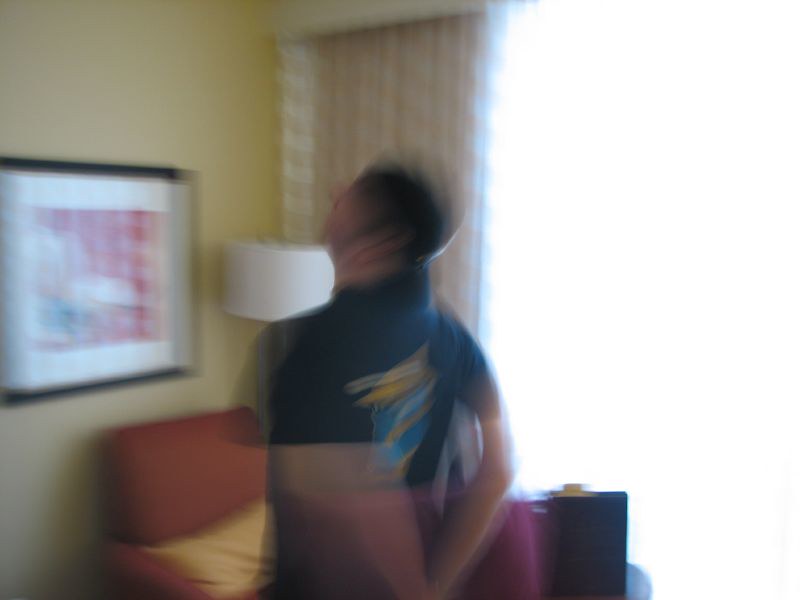A blurry photograph captures a person, likely a man with short brown hair, standing in a room that could be either a hotel room or a formal living room. The individual is wearing a short-sleeved t-shirt, which appears to be blue or black with a graphic print on the back, and has his arms clasped behind his back. The wall is a light buttercup or mustard yellow and features a large piece of artwork with a black or brown frame, a white matting, and a predominantly red print that reflects light, making it difficult to see clearly. To the left of the person, there is additional furniture including a rust-orange chair with a yellow pillow and a reading lamp with a white lampshade. On the right side, an intense white light likely from a window blows out the image. White curtains with a possible red print add to the décor, and a dark rectangular shape, possibly a desk, is also visible in the background.